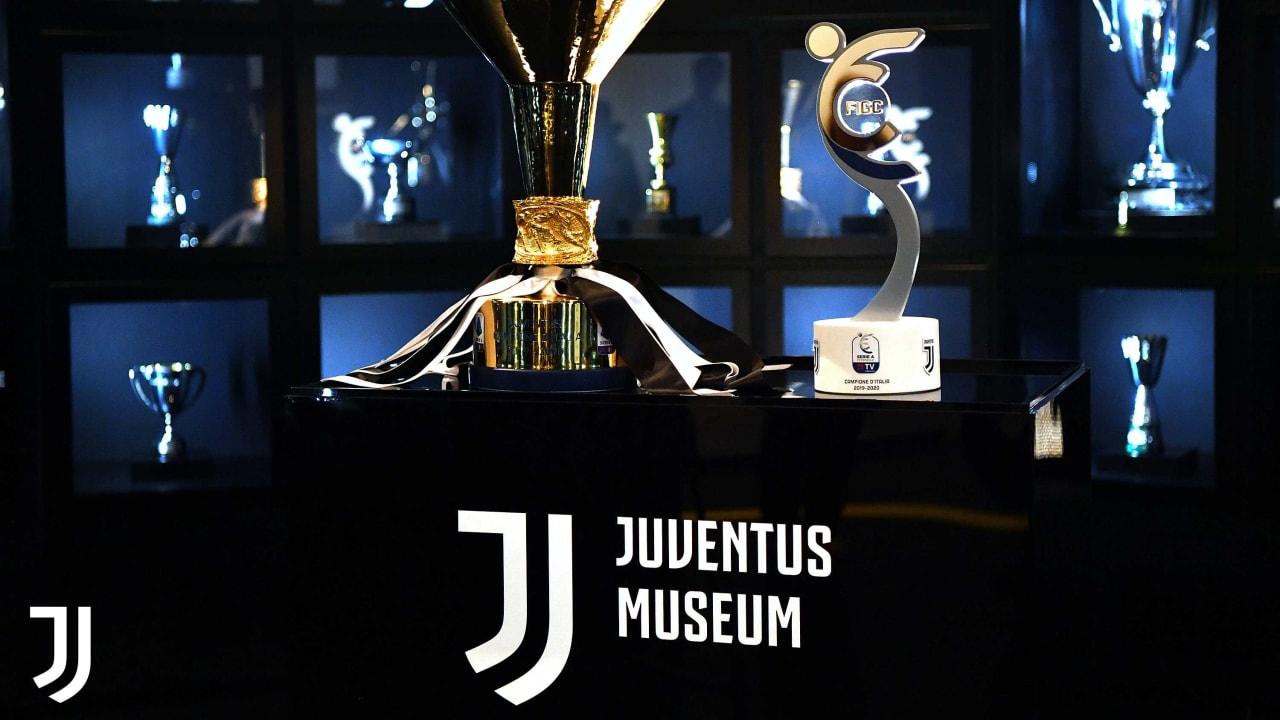The image showcases an award display in what appears to be a museum setting, specifically the Juventus Museum. Dominating the scene is a large, heavy-looking gold award resembling an inverted funnel, supported by feet at the bottom. This prominent trophy sits atop a substantial black box. Accompanying it is a lucite award accented with gold strips and a plastic base. In the backdrop, there is a series of shelves behind glass, each housing various blurred-out trophies. The display area is characterized by a mélange of colors including white, black, silver, blue, brown, and green, with light reflecting off the awards, highlighting their glossy finishes. The overall arrangement of the objects is somewhat haphazard, with some elements extending beyond the edges of the image. The text "Juventus Museum" is prominently displayed at the bottom in large gold letters.